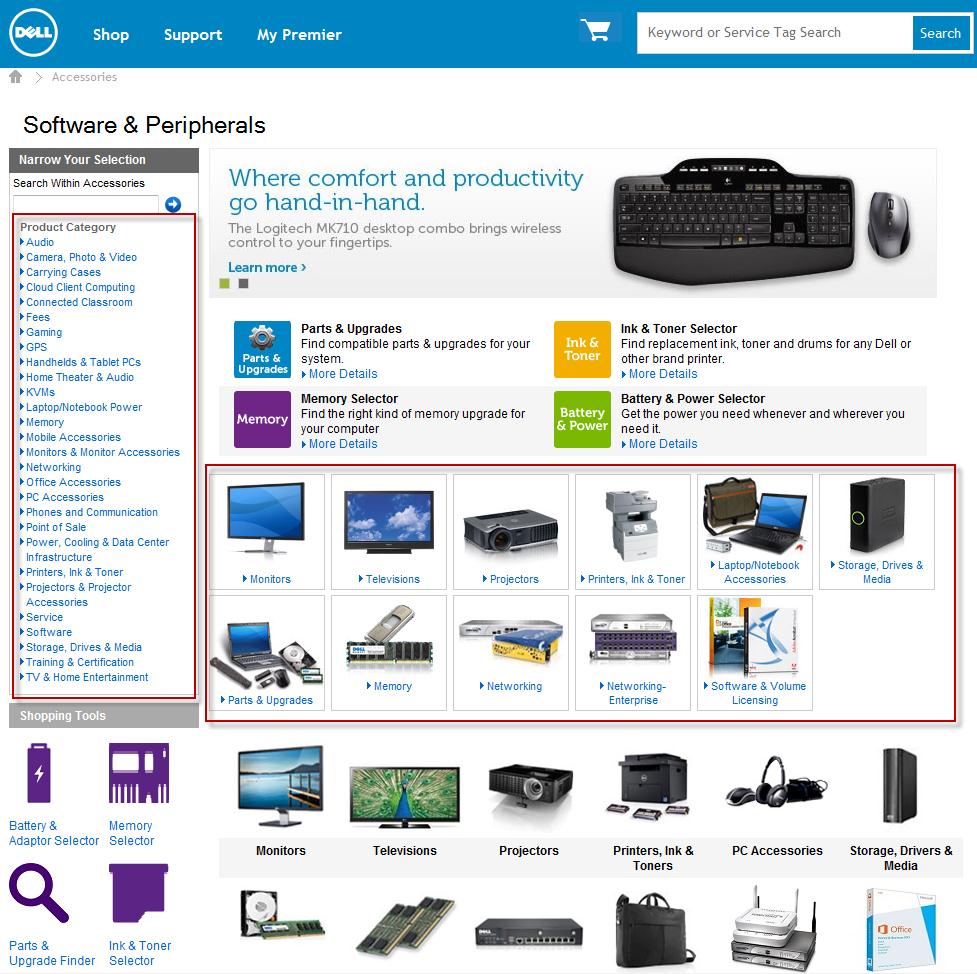A detailed screenshot encapsulates a Dell Computers purchasing page. At the top, a sleek blue Dell menu bar features the Dell logo, menu options for "Shop" and "Support," a partner access point, a cart icon, and a comprehensive search bar that accepts keywords, service tags, or codes. Dominated by a clean, white background, the main content area focuses on the "Software and Peripherals" section.

On the left, a navigable column presents various menus designed to refine your search, listing multiple product categories from "Audio" to "TV and Home Entertainment." This column is distinctly highlighted with a red box outline, suggesting it may serve as a reference or instructional guide.

To its right, the layout showcases an enticing advertisement for a Dell keyboard and mouse, complete with product imagery. Below this banner, several interactive tiles represent different functionalities – from “Parts and Upgrades” to “Ink and Toner.”

Further down, the page prominently displays icons and photographs associated with potential purchase categories, such as monitors, televisions, projectors, printers, and networking equipment. These tiles, also accentuated with red box highlights, facilitate easy navigation and selection.

At the page's bottom, practical "Shopping Tools" include categories for batteries and memory, parts, ink and toner, along with an additional set of photo tiles. Despite their reiteration beyond the highlighted section, these duplicated tiles appear to serve the same purpose, possibly for enhanced visibility or ease of use.